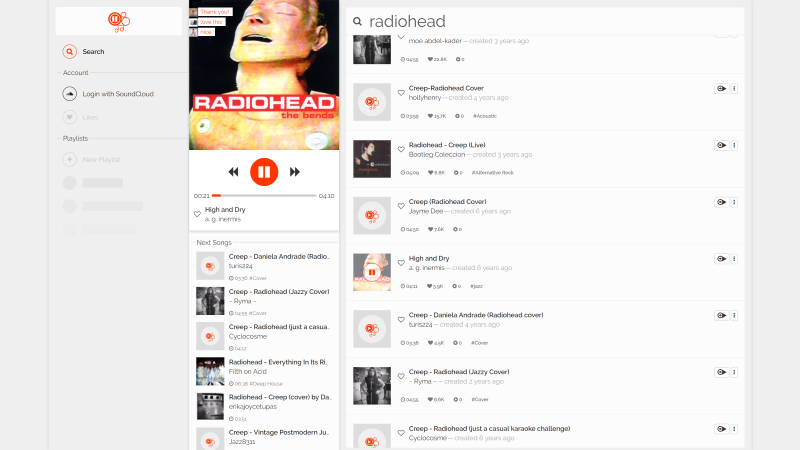**Caption:**

The image depicts a detailed and vibrant webpage interface, primarily featuring light gray backgrounds with solid white menus, accented by dark gray and bright orange elements. 

On the left-hand side, there is a vertical menu. At the top of this menu, within a white rectangular box, sits an orange circular logo featuring a white pause symbol. Directly below, an orange circular button with an orange magnifying glass is paired with bold black text reading "Search." Following this, smaller black text reads "Account."

Further down the menu, two additional icons are observed: one, a black cloud design inside a circle, and the second, a light gray heart shape within another circle. The cloud icon is labeled "Login with SoundCloud," while the heart-shaped icon is accompanied by light gray text reading "Likes." Continuing down the menu, additional text includes "Playlists" and a circular button with a plus sign is labeled "New Playlist."

To the right of this menu is a large, square album cover image. The cover features a humanoid robot's head and shoulders, with closed eyes, detailed facial features, and partial visibility of the neck and shoulder blades. Superimposed over this image is a red box with white text reading "Radiohead," and below it, white text reads "The Bends." 

Beneath the album cover, centered, is a large orange play button flanked by back and forward buttons. Below this play button is a list of text featuring track titles, including “High and Dry,” “Creep,” “Daniela Andrade," "Radiohead," and various covers and versions of “Creep.”

In the main center section of the webpage, there is another vertically oriented list. At the top of this list, large gray text reads "Radiohead" beside a magnifying glass symbol. On the left side of this list are several small square icons of album cover photos. Each album cover photo is aligned with bold titles reading: "Creep," "Radiohead Cover," "Creep Live," "High and Dry," "Daniela Andrade," "Radiohead Jazzy Cover," and "Just a Casual Karaoke Challenge."